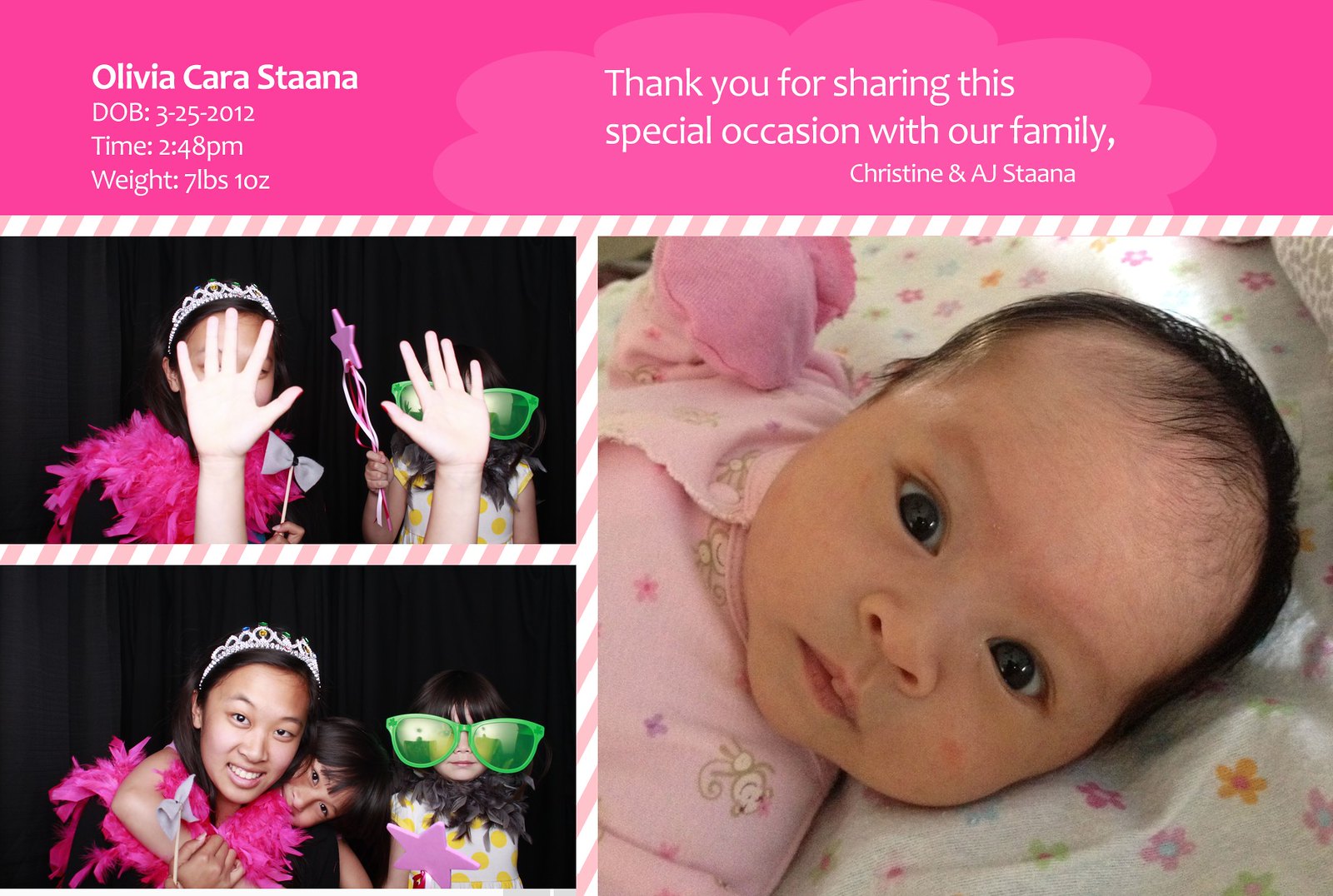The image features a thoughtfully designed birth announcement card. At the top, a pink banner displays key details: "Olivia Cara Stana, Date of Birth: 3-25-2012, Time: 2:48 PM, Weight: 7 lb 1 oz. Thank you for sharing this special occasion with our family, Christine and AJ Stana" written in white print. Beneath this banner, a white border with pink diagonal stripes provides a subtle separation.

The lower portion of the card is divided into three photographs. On the right, a large photo showcases a baby with big dark brown eyes, dressed in a pink outfit with mittens sewn in, laying on a flowered white blanket with its head turned left, showing a hint of black hair. On the left, there are two smaller images. The top-left photo captures two girls posing; the girl on the left wears a tiara and a pink boa over a black outfit, while holding a wand, and the girl on the right sports long dark hair, oversized green glasses, and an outfit adorned with yellow polka dots. In the bottom-left image, the same two girls are joined by a third, younger girl positioned between them, tilting her head to the right and touching her mouth on the pink boa. The girl with the green glasses holds a purple star accessory.

The color palette of the card includes various shades of pink, white, tan, green, yellow, and black, contributing to the overall warm and celebratory feel of the announcement.